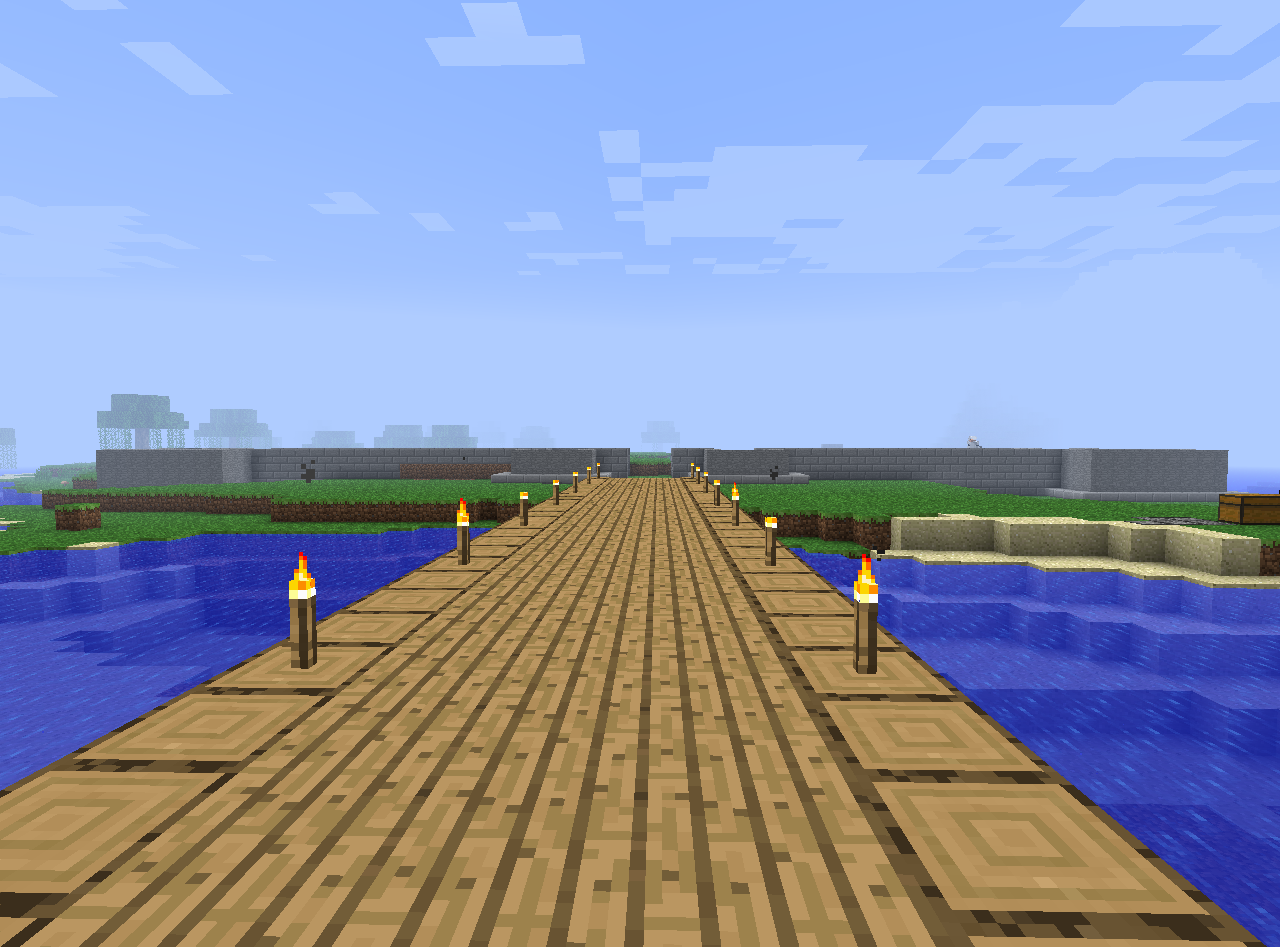This computer-generated image is a square composition that features a serene and aesthetically pleasing scene. The backdrop showcases a gradient sky, transitioning from a light blue at the horizon to a deeper blue above, peppered with lighter blue patches that suggest an artistic interpretation of clouds. Dominating the foreground is an elongated wooden dock, adorned with brown poles that support strategically placed lights, casting a soft illumination over the scene.

The dock extends over a body of water, which appears to be a dark, rich blue accentuated with light blue highlights that create a sense of movement and reflection. The water's edges form triangular shapes around the base of the poles, adding to the geometric harmony of the image.

To the left of the composition, there is a lush patch of greenery. A small hill, draped in green grass with earthy brown patches, gently rises from the green expanse, adding depth to the landscape. A gray brick wall forms the backdrop, spanning across from left to right, with an opening at the end of the dock hinting at a passage or further scenery beyond the frame.

The meticulous details in color and structure evoke a tranquil, almost dreamy atmosphere, blending the natural and constructed elements seamlessly.